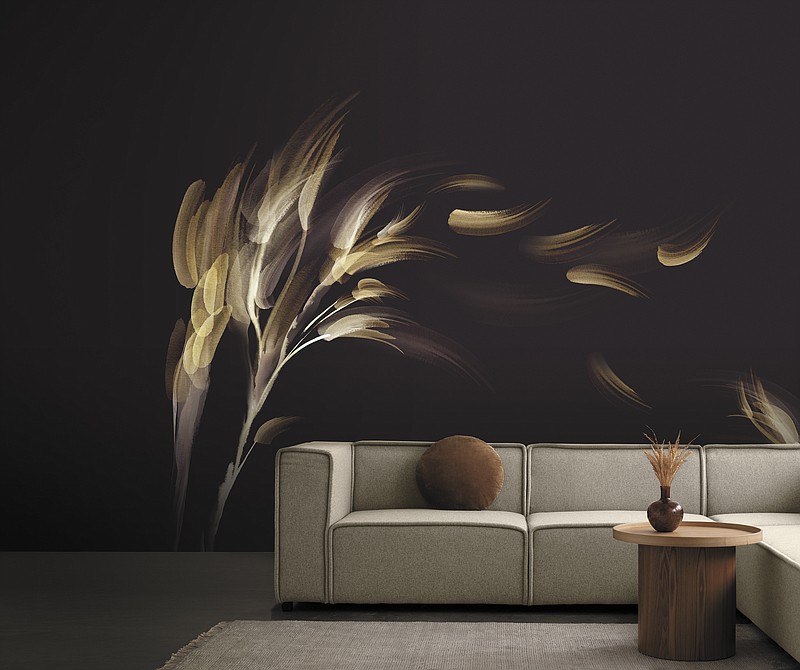This striking modern living room features a sophisticated gray sectional modular sofa adorned with a round brown velvet throw pillow. Positioned in front of the couch is a unique coffee table that resembles a wooden log, topped with a circular tray holding a brown ceramic vase filled with dried grasses. The sofa rests on a gray area rug, which partially covers the room's darker gray-tone flooring. The backdrop is a bold black wall mural, artistically decorated with an abstract depiction of feathers or wheat stalks being blown by the wind, rendered in graphic detail with brown highlights. The overall aesthetic is contemporary and stylish, making it an appealing space for those with a taste for modern, abstract design.